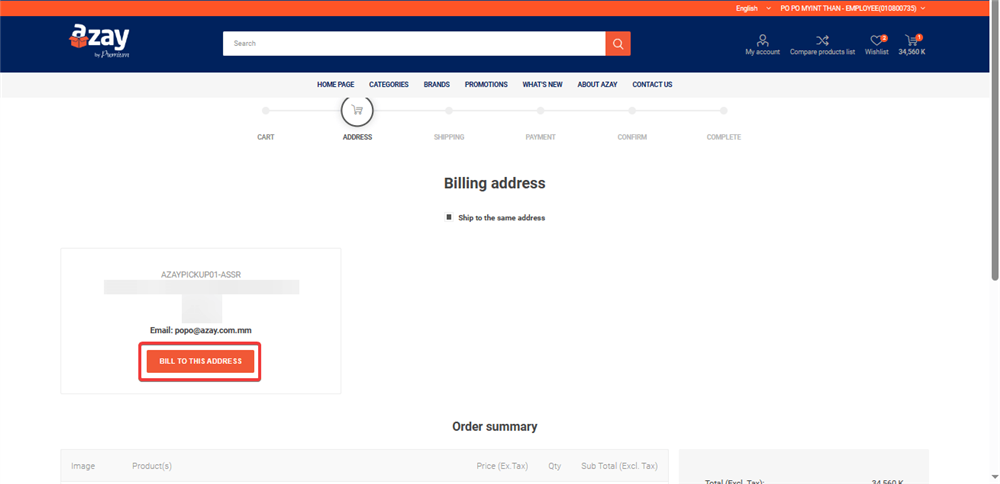A screenshot of a web page from a bulk seller platform, Azay. The website features a white search bar at the top followed by an orange navigation bar that shows options for English language selection, employee ID, account details, comparison list, and wish list, which has two items. The cart shows one item priced at $34,560k. Below the search bar, there are blue-on-white navigation options for the homepage, categories, brands, promotions, what's new, information about Azay, and contact details. A clear order process line is displayed, indicating cart, address, shipping, payment, confirmation, and completion steps. The screenshot highlights the billing address, encased in an orange box surrounded by a red circle on the bottom left, along with a code labeled ASSR, and an email contact. The order summary and specific product details are partially cut off, but the page resembles a functional, bulk-purchase online store similar to Amazon, likely targeting an Asian market.